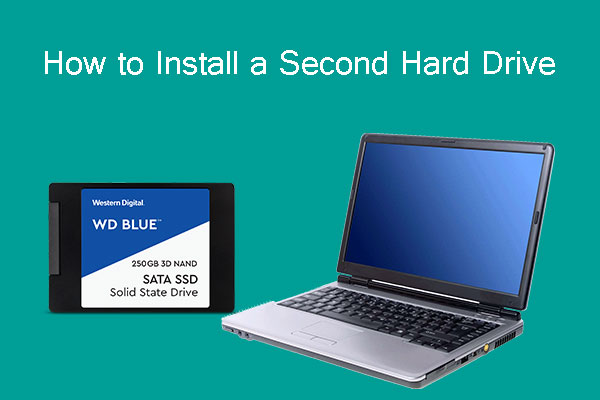The image is an instructional diagram on a teal blue background, titled "How to Install a Second Hard Drive" in prominent white text at the top. It features a laptop with a silver base, a black frame around the screen, and a black keyboard. The laptop's screen displays a blue gradient transitioning from dark blue at the bottom left to lighter blue at the top right. To the left of the laptop, there is a solid-state drive (SSD) shown head-on as a black rectangle. The SSD's label has a blue section on the top left that transitions diagonally to a white section on the right. The label displays "Western Digital WD Blue" in white text on the blue background and "250 GB 3D NAND SATA SSD Solid State Drive" in black text on the white background. The SSD image is an inset and appears disproportionately large compared to the laptop, suggesting it is a separate element intended to highlight the specific hard drive model required for the installation process.